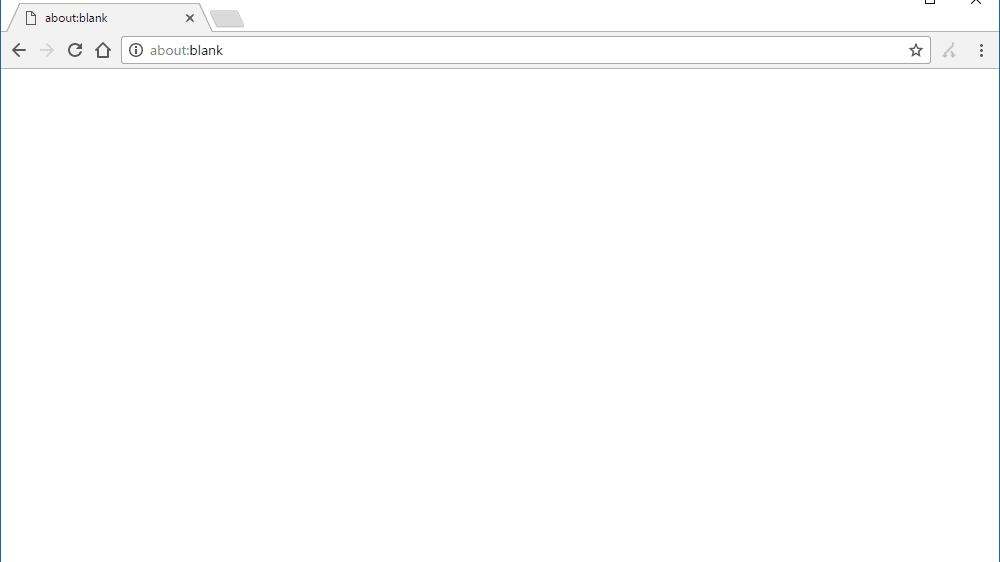The image depicts a completely blank web browser screen with a white background. At the top of the page, the address bar reads "about:blank." To the left of the address bar, there is a black arrow pointing to the left, signifying the back button. Next to it, a grayed-out arrow pointing to the right indicates the forward button. The toolbar also includes a circular arrow for page reload, followed by a home icon. On the right end of the address bar, there is a star icon for bookmarking and an icon of three vertical black dots, representing the browser's menu for additional options. The screen is devoid of any photographic elements, people, animals, plants, buildings, vehicles, or any other objects or structures. It is an entirely empty browser interface displaying no content.